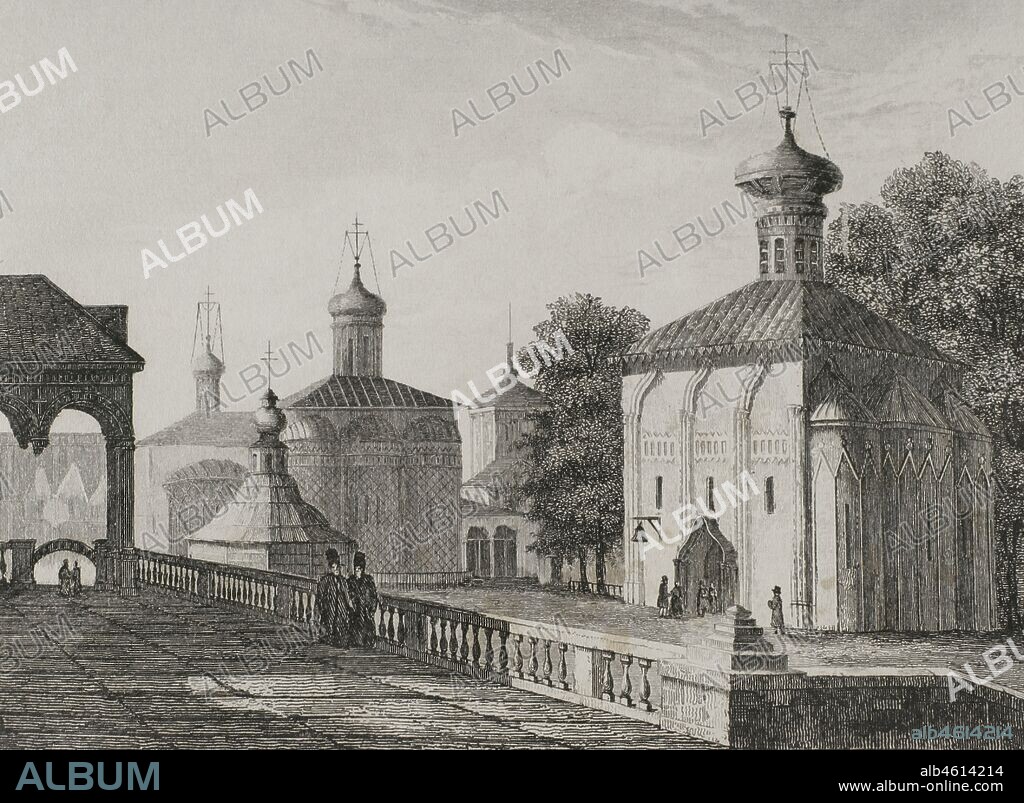This black-and-white illustration, reminiscent of an old textbook drawing, captures a scene filled with architectural and human details. The bottom of the image features a black rectangle: on the bottom left, the word "Album" is written in light blue, while on the bottom right, "ALB4614214" and "www.album-online.com" are noted. A watermark of the word "Album" appears repeatedly across the image, likely as a copyright measure.

The central subject of the artwork is a series of buildings with a distinctly old Russian aesthetic, characterized by bulbous spires and crosses, indicating that they are likely churches or ecclesiastical structures. The buildings are small and squarish, with curved chimneys extending up to cross-topped steeples. In the background, there are trees and a sky filled with clouds.

In the foreground, to the left, there's an area that resembles a wooden tiled space surrounded by a fence. Overlaying this area, a sort of bridge or footbridge extends, on which two individuals in long black coats and tall black hats can be seen walking. Scattered throughout the image are numerous figures – at least nine – dressed in period attire, going about their daily activities, adding a lively touch to this historical scene.